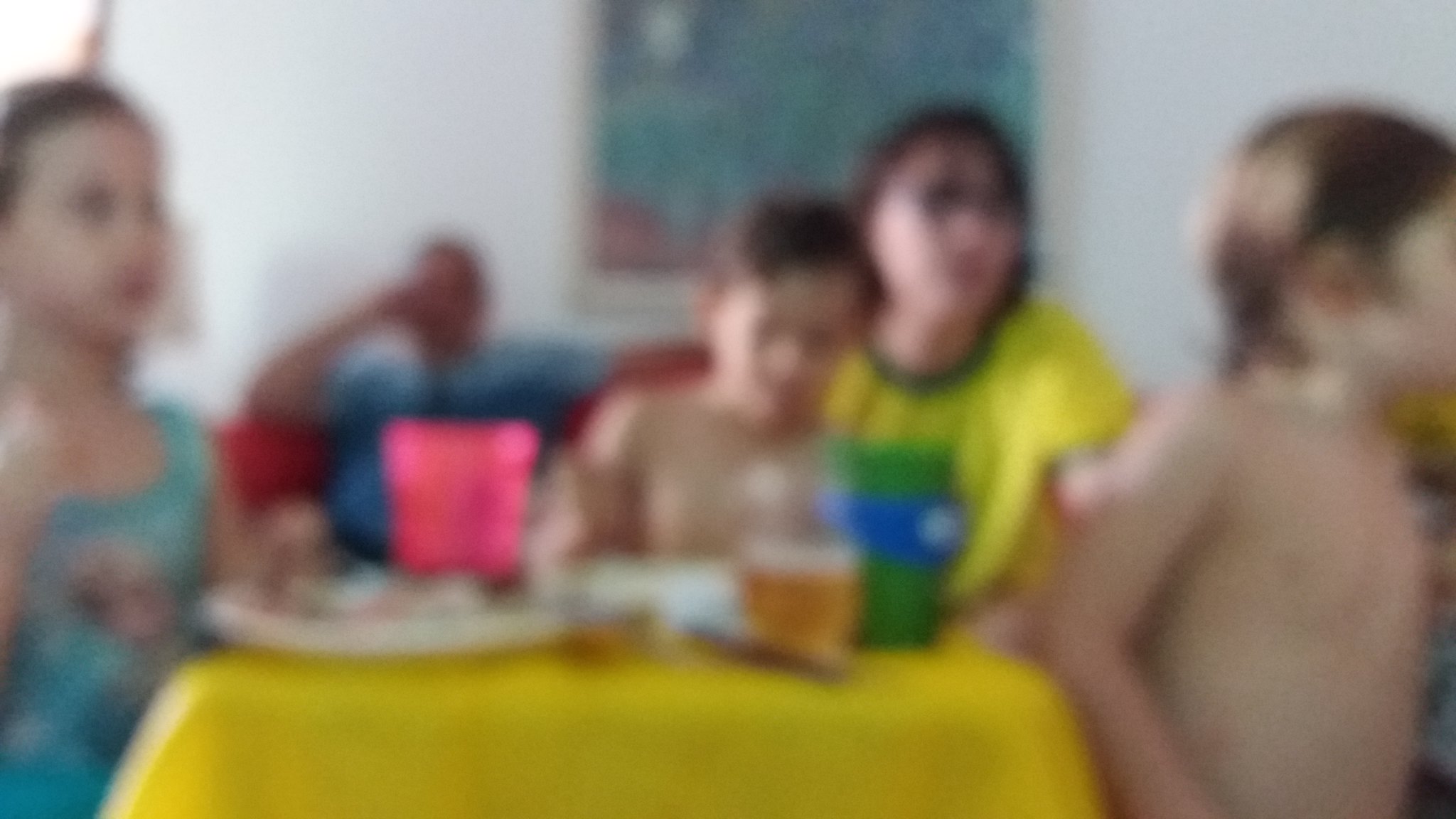This image captures a blurry scene featuring a group of people in what seems to be a casual, possibly poolside gathering. Central to the photograph are four individuals: three children and one teenager or slightly older person, sitting around a small table covered with a yellow tablecloth. The table holds a few items, including a pink plastic cup and a green plastic cup with a blue band, along with some plates. 

On the far left, there is a young girl or perhaps young teenager in a leotard or swimsuit, which appears to feature a design of Elsa from Frozen, though the image's blur makes it difficult to confirm. Directly behind the table, a young boy without a shirt is visible. He might be seated in front of or on the lap of an older person who wears a yellow t-shirt with a green collar. This person has dark hair and may be wearing glasses. To the right, another shirtless young boy is seen, suggesting they might have just been swimming or attending a pool party.

In the background, another individual is seated on a red couch. Above this person, there is a framed painting or a window on the wall, further adding to the casual, home-like atmosphere of the scene. Despite the blurriness, the image conveys a moment of relaxed, likely summer-time enjoyment among the group.